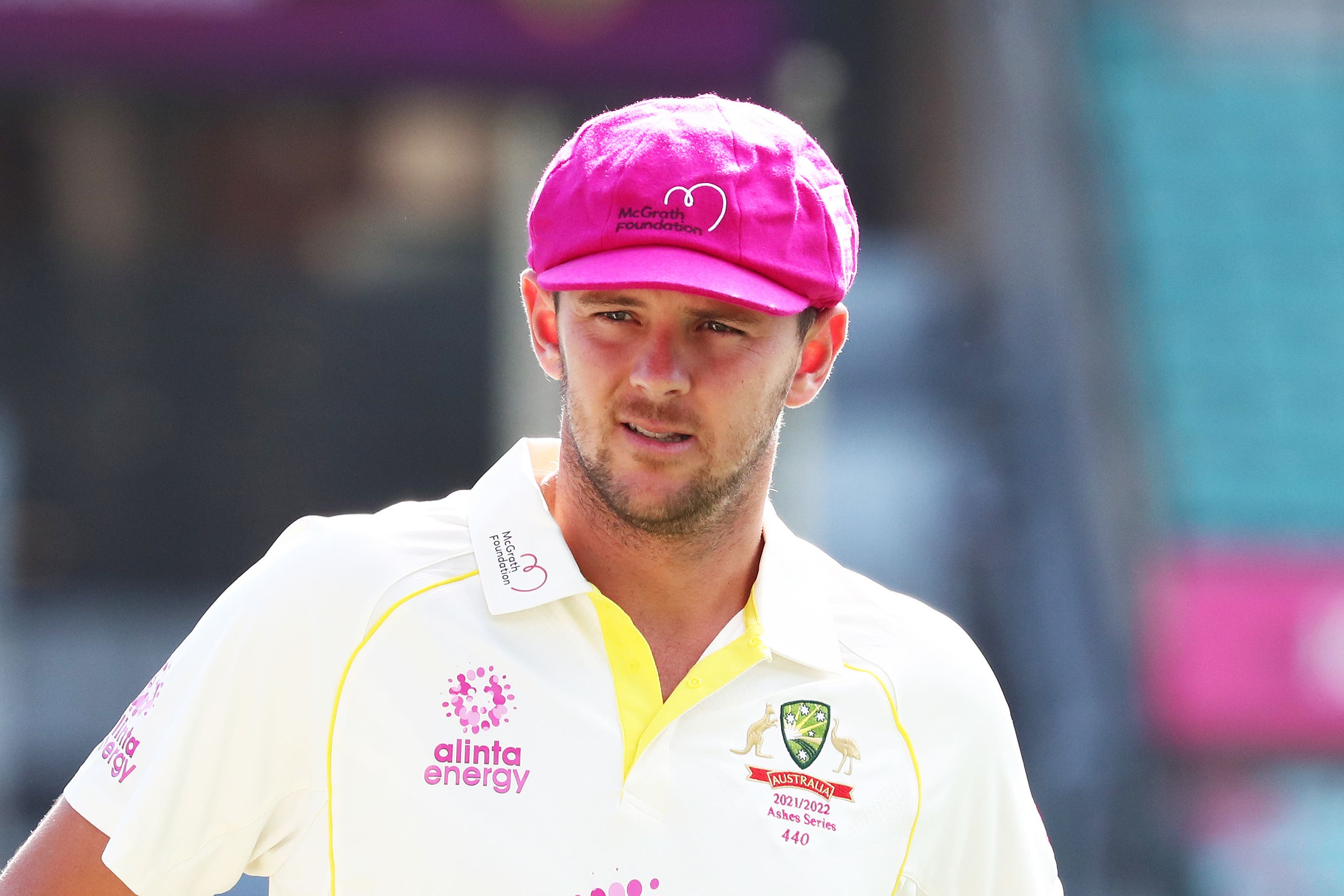The photograph features a Caucasian male engaged in a sporting activity, possibly cricket, signified by his attire and surroundings. He wears a bright pink baseball cap emblazoned with "McGrath Foundation" and a stylized half-heart graphic in black. His white polo shirt is accented with yellow piping around the collar and down the sides of the arms. On the left side of his shirt (from the viewer's perspective), there's a pink burst with "Alinta Energy," a visual mirrored on his left sleeve. The right side of his shirt bears the emblem "Australia 2021-2022 Ashes Series 440," accompanied by a shield flanked by a kangaroo and an emu, which contains a green patch with a sun and stars. Additional "McGrath Foundation" text, along with the heart motif, also appears on his collar. The man is smiling towards someone outside the frame to the left, and he's sporting facial hair, including a beard and stubble.